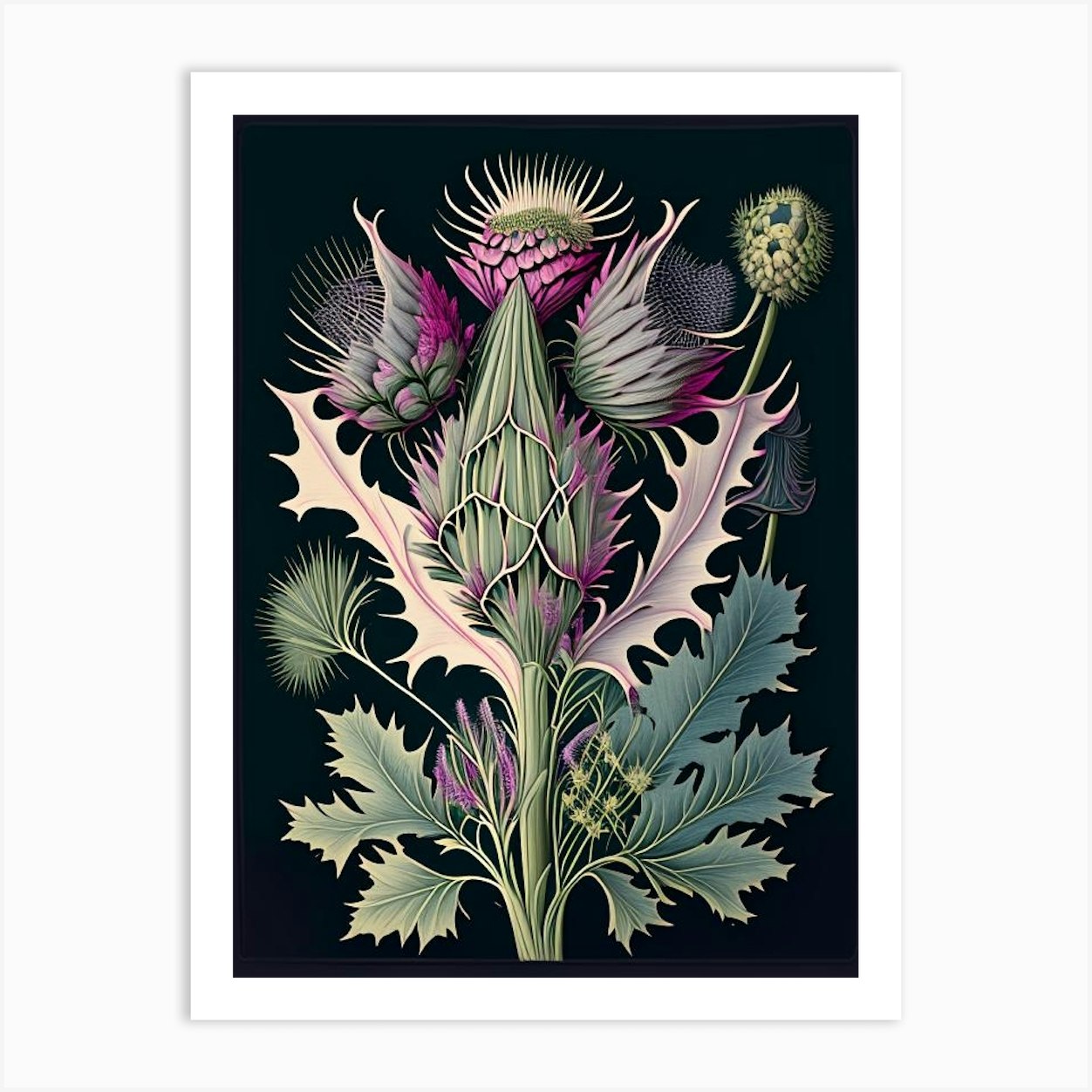This is a detailed illustration of a fantastical plant, set against a black background with a thin white frame. The main central stem of the plant extends upward from the bottom, curving gracefully to form a prominent green bulb adorned with purple spikes at its apex. Dark green serrated leaves extend asymmetrically from the stem, interspersed with both yellow and purple flowers. High above the main bulb, the plant features additional purple spiky leaves - one jutting out to the right and another to the left. Crowning the central bulb are four smaller bulbs, three of which are similar in size and exhibit a mix of gray, pink, and yellow hues. The fourth, positioned on the right, is smaller and distinctly yellow. Various spiky seed pods can also be seen attached along the length of the stem, adding to the plant's otherworldly appearance. Overall, this artwork presents a highly detailed and imaginative depiction of a plant that blends vibrant colors with a strikingly bold composition.